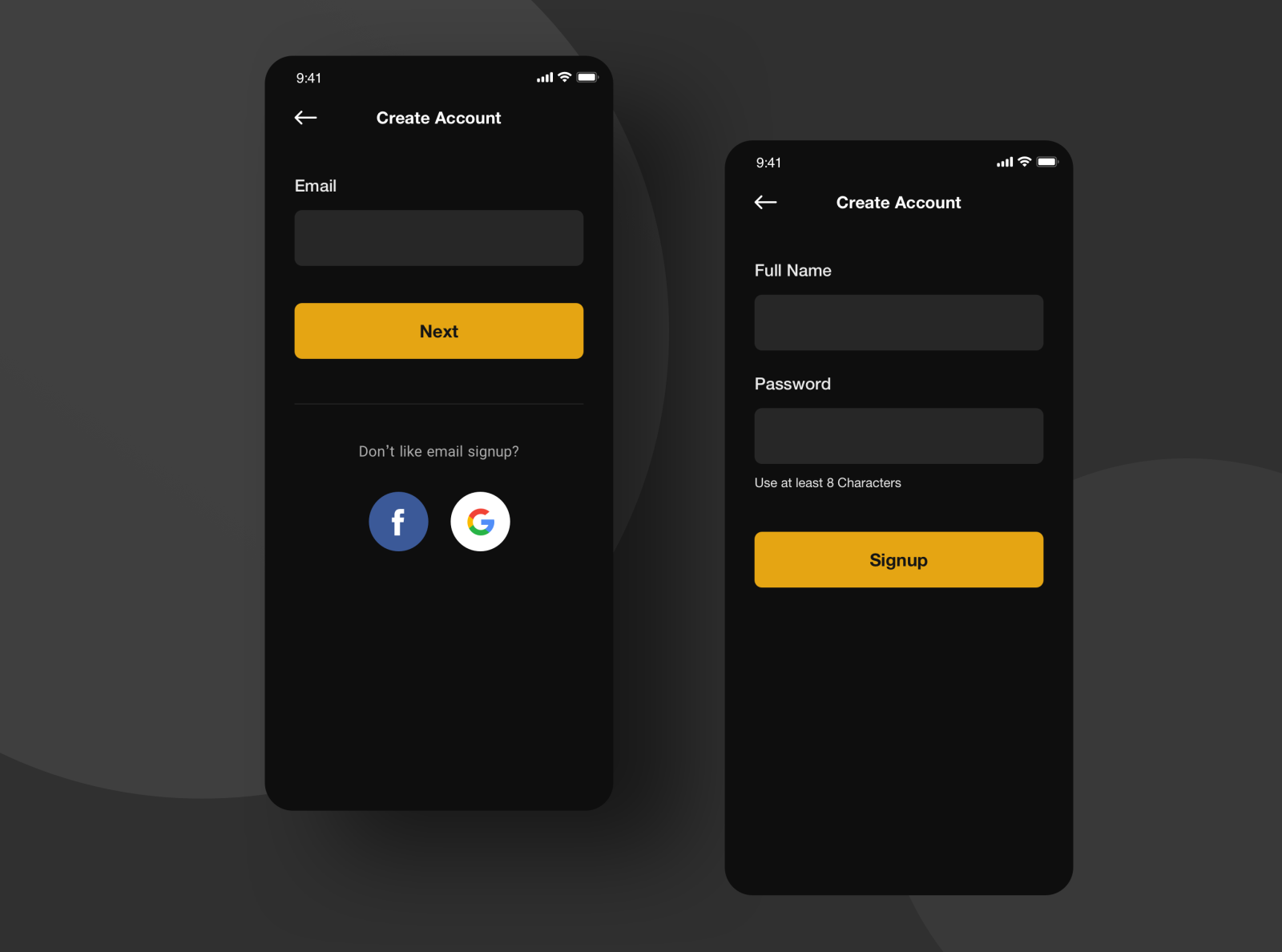The image is a detailed screenshot showcasing the "Create Account" sections of a registration process. On the left side of the screenshot, there is a "Create Account" header at the top. Directly below the header, there is a field labeled "Email" with a corresponding text box for input. Beneath the email field, an orange button with the text "Next" is prominently displayed. Below this button, there is a phrase "Don't like email sign up," followed by two circular icons: the Facebook logo on the left and the Google logo on the right for alternative sign-up options.

The right side of the screenshot continues the "Create Account" process with a header at the top. This section has text fields for "Full Name" and "Password." There is an instruction below the password field that reads, "Use at least eight characters." At the bottom of this section, there is a "Sign Up" button. This comprehensive layout demonstrates various stages and options for account creation.